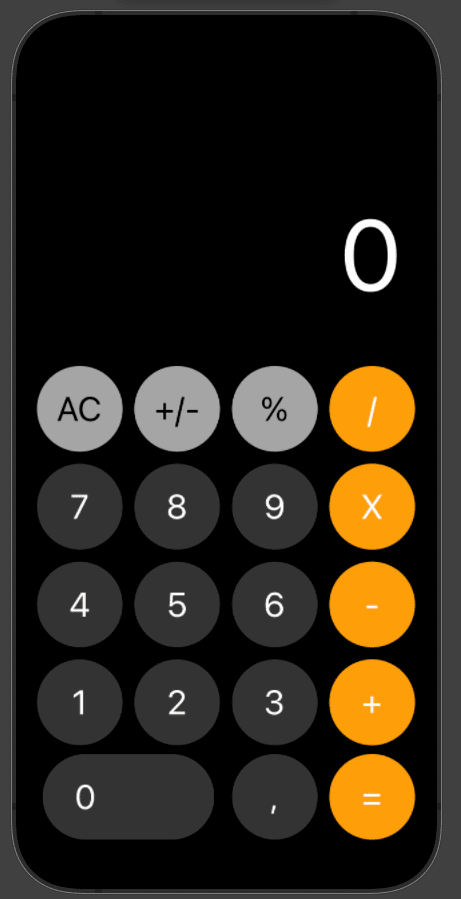The image features a vertically rectangular frame showcasing a close-up view of a smartphone screen with rounded corners. Set against a pitch-black background, the phone's calculator app is open. At the top portion of the screen is a large black display area with a single white zero aligned to the right. Below this display, the calculator keys are arranged in a grid. The keys for functions 'A', 'C', positive/negative conversion, and percentage are circular and shaded in a medium gray tone. The vertical series of keys for division, multiplication, subtraction, addition, and the equal sign are distinctly highlighted in bright orange. Completing the layout, the numeric keys from 0 to 9 and the decimal point key are colored in a dark gray, adding contrast and delineation to the interface.